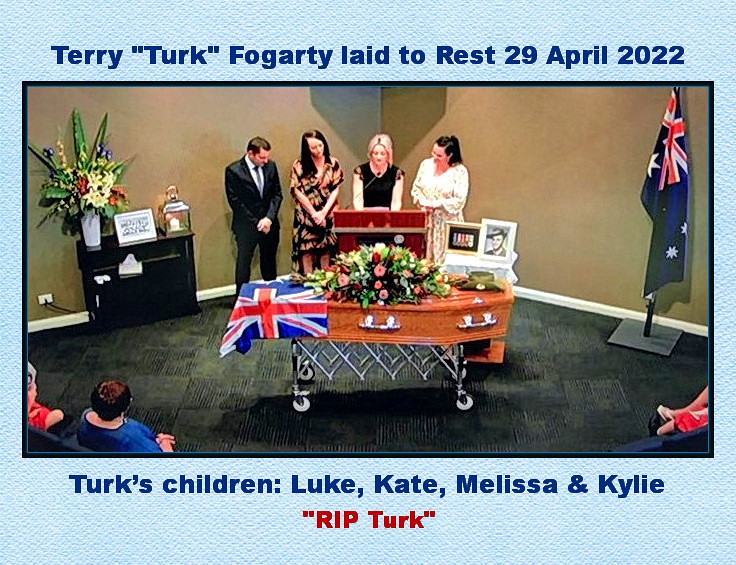The image depicts a solemn indoor funeral setting, prominently featuring a wooden casket adorned with a large array of flowers and draped with a British flag on the left-hand side. Beyond the casket, there are framed photos of the deceased, Terry Turk Fogarty, alongside some military medals. The right-hand corner showcases another British flag on a stand. Four people, identified as Terry's children—Luke, Kate, Melissa, and Kylie—stand behind a podium situated behind the casket. They are wearing appropriate funeral attire, with one of the women speaking into a microphone. To their left, there is an arrangement of flowers and a black stand with a box of tissues. In front of this setup, attendees are seated, listening to the speakers. The image has a blue patterned background and a blue header reading "Terry 'Turk' Fogarty, laid to rest 29 April 2022," with a bottom note stating "Turk's children, Luke, Kate, Melissa, and Kylie, Rip Turk." The overall scene reflects a moment of tribute and remembrance for the deceased.